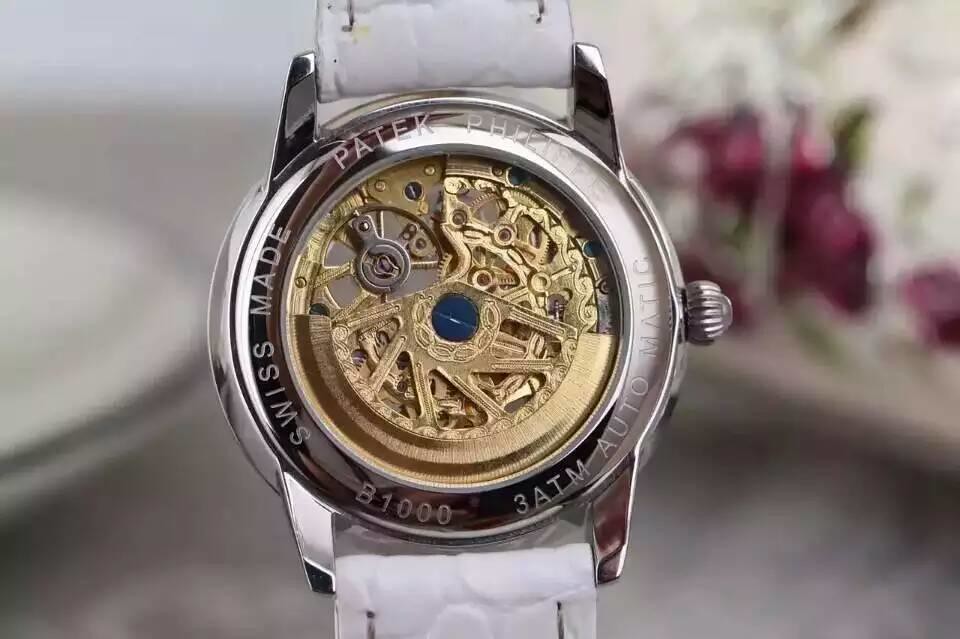A close-up image showcases an intricately designed wristwatch with a prominent white wristband, which appears worn and slightly dirty. The watch features a silver knob on its side and a distinctive silver bezel engraved with a series of letters and numbers. The intricate inner workings of the watch, highlighted in gold, are partially visible through a small corroded dark blue circular component at the center. Off to one side, there is a smooth, rounded silver portion adding to the watch's aesthetic. In the background, a blurred purple and green object provides a contrasting backdrop, while a hint of light reflects off the silver elements of the watch, emphasizing the excellent quality and clarity of the image.